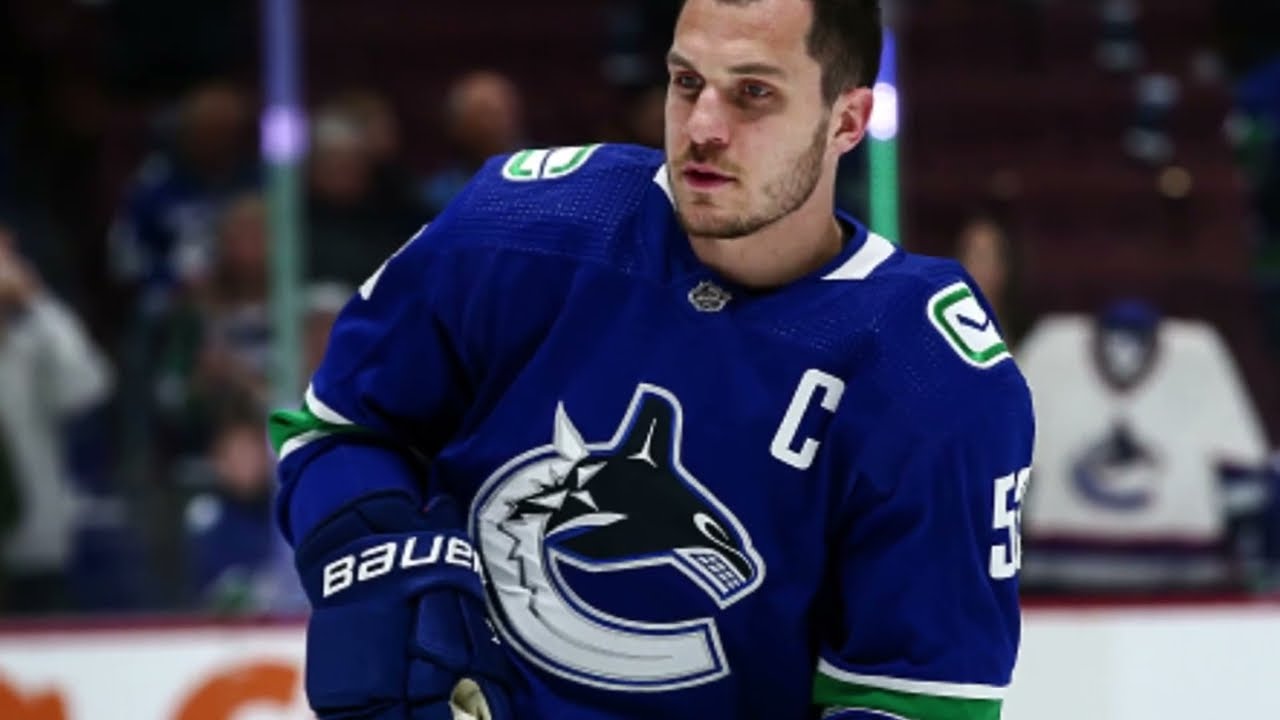This is a detailed photograph of a Caucasian male hockey player with dark brown hair, a trimmed beard, and mustache, on the ice rink. He is wearing a royal blue jersey featuring a prominent white letter 'C' on the upper left chest, signifying his captaincy. The front of his jersey displays the head and dorsal fin of an orca, which is black and white, emerging from the middle of the letter 'C'. His right-hand glove, colored blue, bears the brand name "Bauer" in white lettering. Part of his uniform number, potentially '53', is visible on his sleeve. The background shows a blurred stadium crowd with some spectators and distinctive blue and green pillars. A white jersey identical to his hangs on a piece of glass in the stands, further suggesting the home team's presence. The player is looking to the left, and his lack of a helmet makes his facial features and short-cropped hair more noticeable.